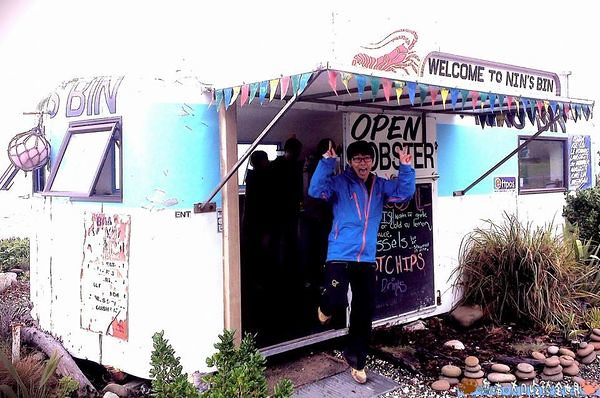In this vibrant outdoor scene, a young man with short, dark hair and glasses is stepping out of a stationary food truck that appears to be set up like a small diner. He is wearing a blue jacket and black pants, with one hand making a V sign while the other points up in the air. His expression is lively and cheerful. The food truck, which resembles an old Airstream with peeling white paint accented by blue stripes, is adorned with colorful flag decorations along its awning.

Prominently displayed atop the truck is a sign featuring a picture of a lobster and the welcoming words "Welcome to Ninh's Bin." To the right of the man, there is an open window where orders are likely taken, and to the left, a small buoy hangs near another window. At the base of the truck, potted plants and shrubs add a touch of greenery, as does a mat upon which the man is stepping. In the background, a blackboard menu lists the items being sold, and a clear sign behind him reads "Open Lobster," signaling that the food stand is ready for business. Rocks and more plants are scattered around the vicinity, enhancing the rustic charm of this unique dining spot.